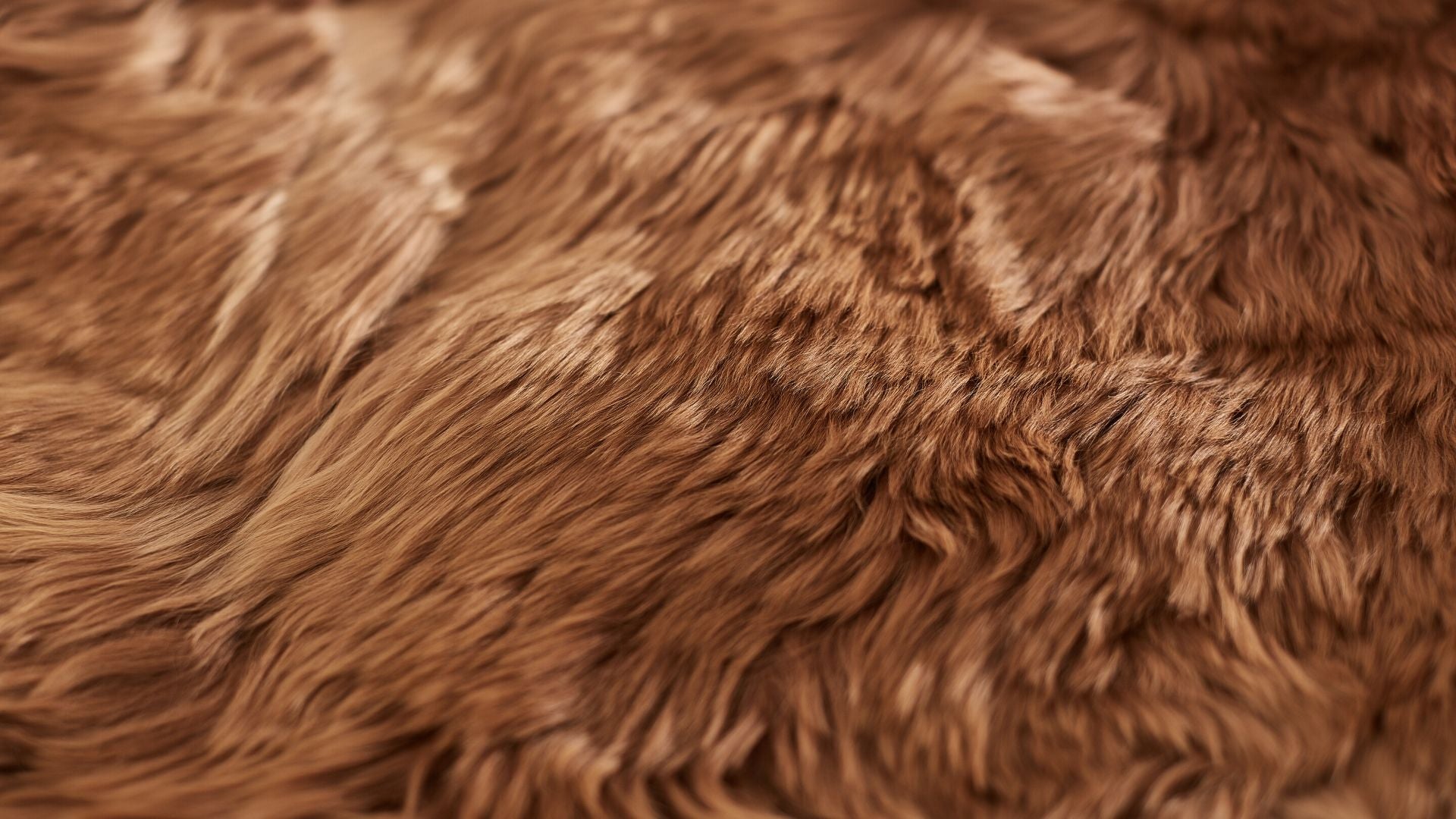This close-up image captures what appears to be a rich, auburn, or reddish-brown texture, reminiscent of either fur or a thick, wavy rug. The texture mimics the flowing, gently waved appearance of an animal's coat, potentially that of a cocker spaniel or golden retriever. The image focuses intensely on the varying lengths and hues, with the left part showcasing a slightly lighter brown color that transitions to darker brown toward the center and bottom right of the frame. The fur—or fabric—encompasses the entire image, filling it with its slightly groomed yet natural, unkempt waves. The focus is sharper in the middle and softer around the edges, adding an additional layer of texture depth and complexity. This ambiguity in texture could suggest fur, a plush rug, or a fuzzy blanket, but the exact material remains indistinct. The detailed, zoomed-in portrayal underscores the softness and waviness, emphasizing the tactile quality of the subject.